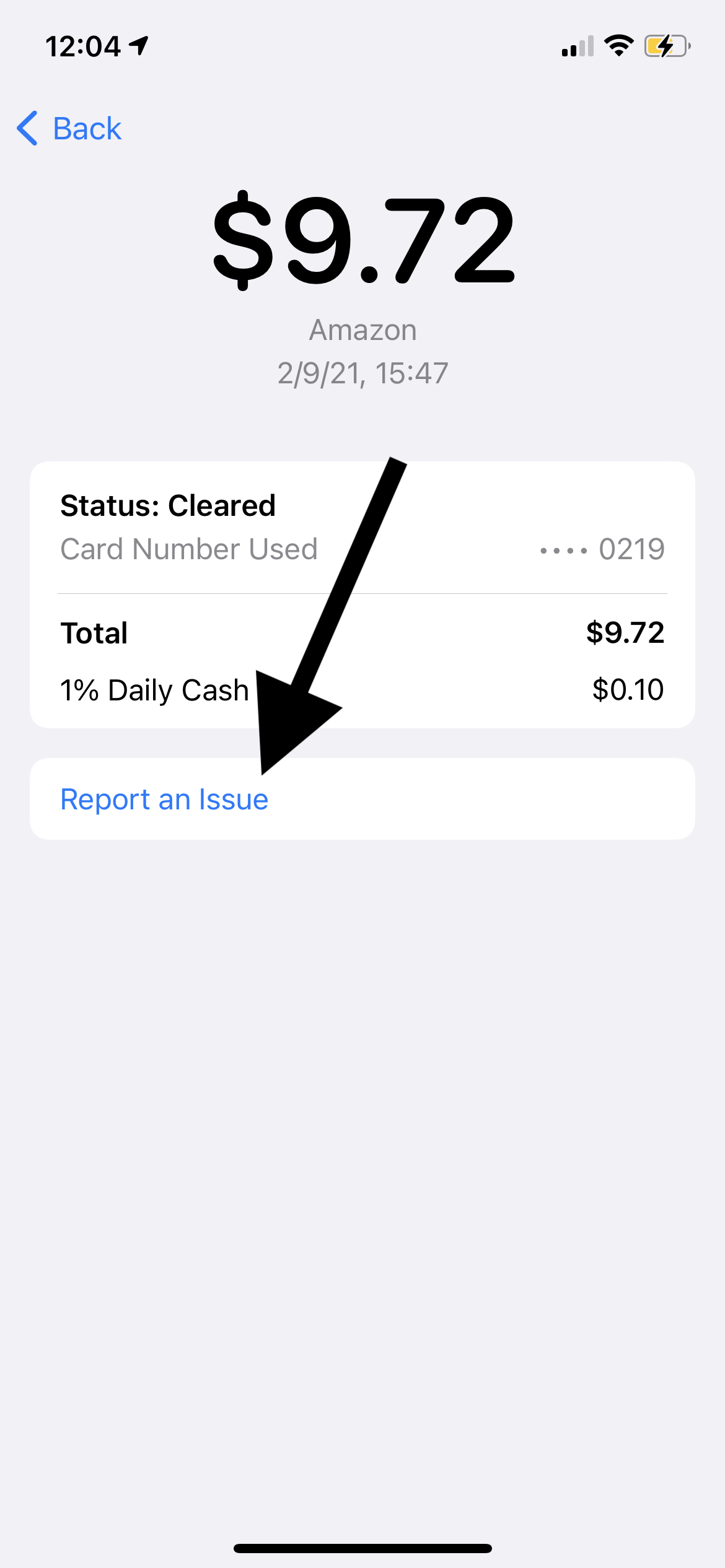The image is a screenshot of a smartphone screen, featuring either an Amazon or a credit card application interface. The background is light gray, and it is 12:04 PM, as indicated by the black time display at the top. The status bar shows a partially filled battery icon and a Wi-Fi signal with two out of four bars.

Centered at the top in large, bold black font is a monetary amount, "$9.72." Directly below, in lighter black text, it reads "Amazon," followed by the date "2921" and the time "15:47."

Beneath this information is a white horizontal box. In the top left corner of this box, in bold black text, it states "Status: Cleared." Below this, in light gray, it reads "Card Number Used," with the last four digits "0219" displayed on the far right.

Further down, also in bold black text, it says "Total 1% Daily Cash." To the right of this, it displays "$9.72" with "10¢" underneath. 

In the bottom left corner of the screen, within a separate white box, there is an option to "Report an Issue" in blue text. A large, bold, diagonal black arrow points to this button, emphasizing its location.